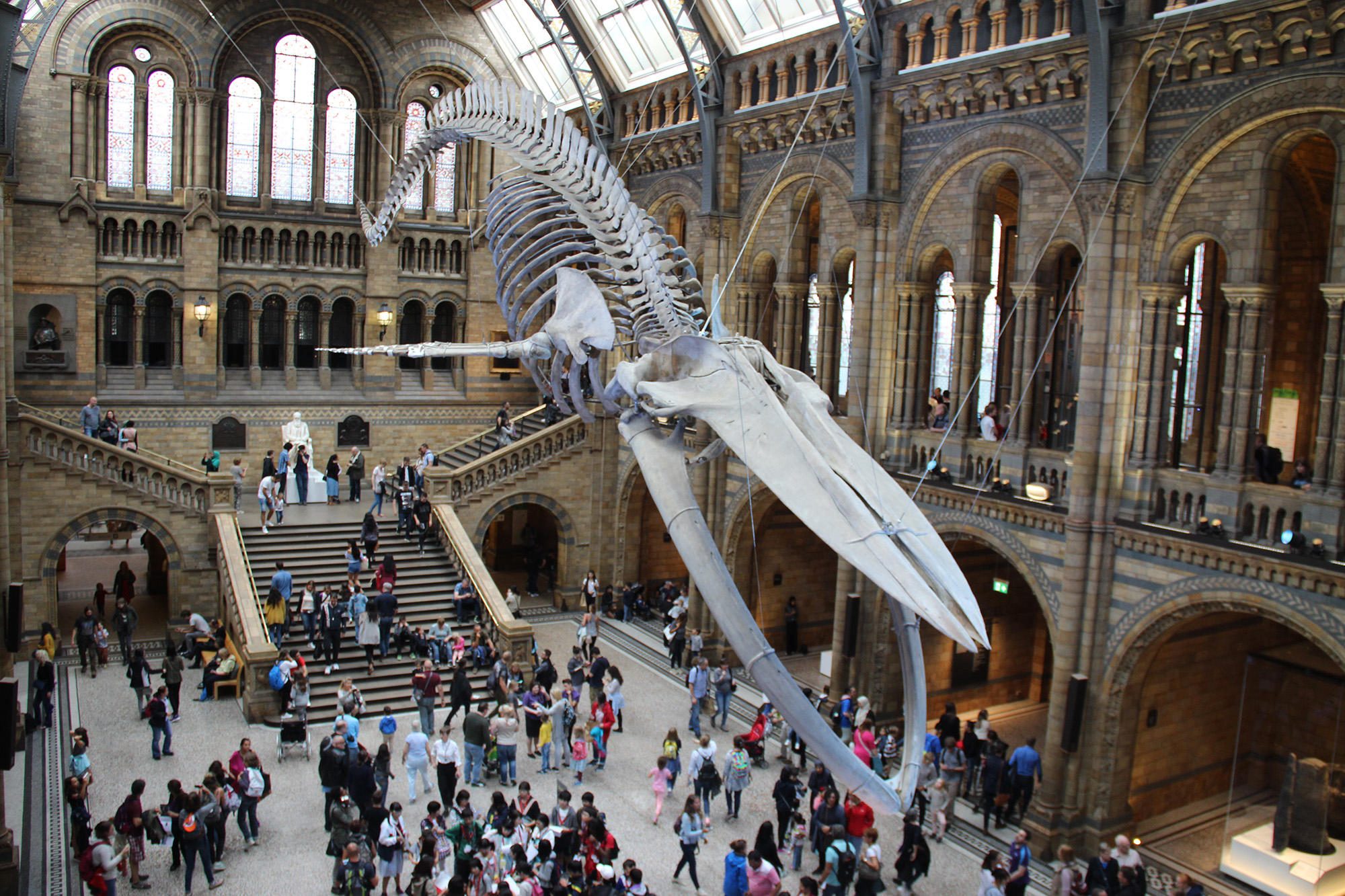In this image of a bustling natural history museum, visitors are seen exploring the spacious and meticulously maintained ground floor. The large open area is crowded with people who are conversing, taking photos, and wandering about to view the exhibits. The museum's architecture is striking, featuring a tall ceiling, light stonework, and numerous archways that give it a cathedral-like atmosphere. Dominating the scene is a massive skeleton of a whale, suspended from the ceiling and seemingly swimming toward the camera with its mouth open. This lifelike display fascinates the visitors below who are scattered and clumped in small groups. A grand staircase with multiple landings, stairways veering left and right, and a marble sculpture on one of the landings, adds to the grandeur of the scene. Natural light floods the room through decorative arched windows and possibly stained glass, illuminating the detailed and historical ambiance that appeals to the throngs of people present.